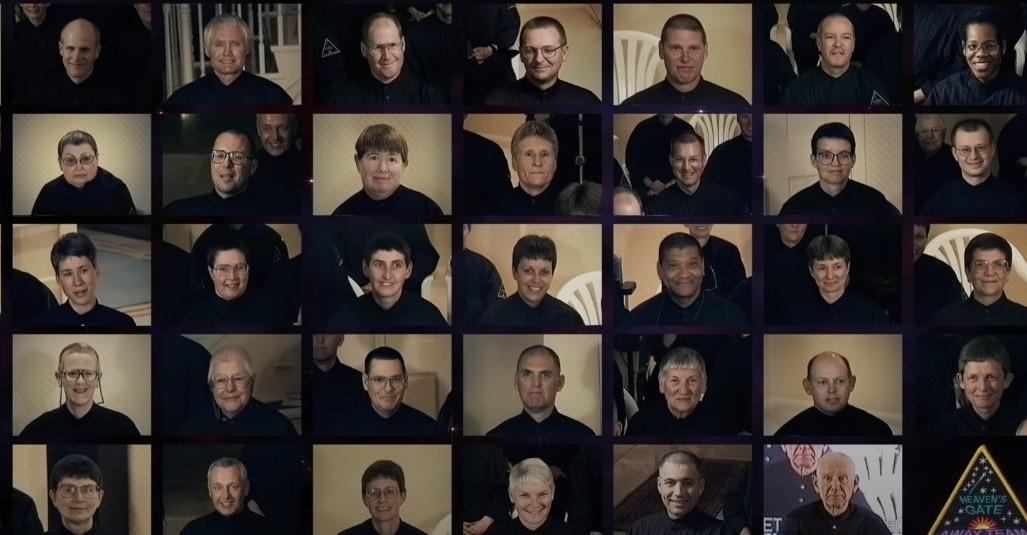This photo appears to be a Zoom-like collage featuring a diverse group of individuals arranged in a grid of small squares with approximately seven across the top row and three to five down. The background is black, emphasizing each person's upper body from the neck up. All participants are dressed in black robes reminiscent of judges, and most have short hair. The top row consists solely of men, largely white with one potentially black individual, while lower rows include a mix of men and women who appear to get younger as the rows descend. The array also shows varying ethnicities, though predominantly white. The bottom right square contains a yellow, upside-down V with light blue letters spelling "GATE" and an image of a rising sun beneath it. There's an implication that these images might have been compiled for a special occasion such as a graduation or a religious assembly, suggested by their uniform attire and the formal presentation of the grid.